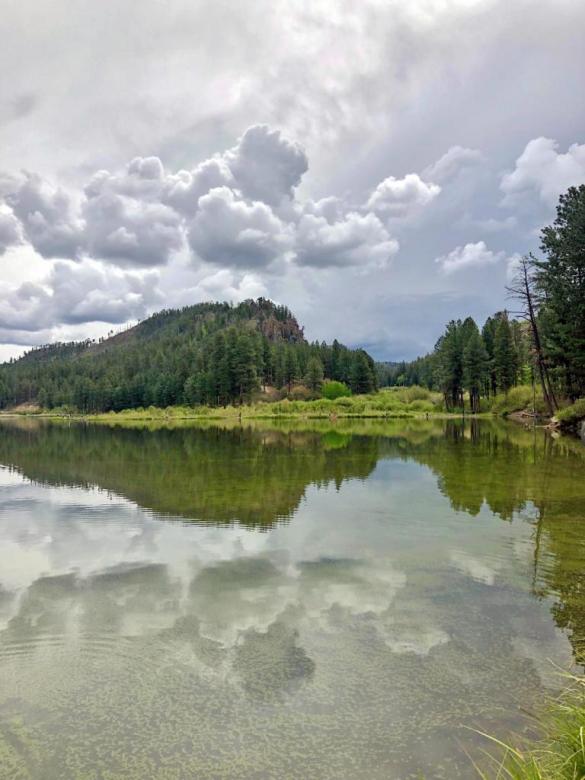This is a detailed photograph of a serene lake set against a large, forested, and mountainous backdrop. The water in the foreground is relatively still, with subtle ripples, and richly reflects the overcast sky, which hints at a touch of blue with the sun trying to peek through the clouds. You can see the intricate reflection of the dense forest, composed mainly of green pine trees, with some color variation in the mirrored image. The surface of the lake shows signs of algae growth and grass near the water's edge, particularly noticeable at the bottom right of the image. The forest itself stretches over a series of mountains and hills, featuring a small valley filled with large, lush trees. The scene conveys a sense of isolation and tranquility, with no signs of human habitation, accentuated by the cloudy sky which is heavier on the left and clears slightly towards the right.